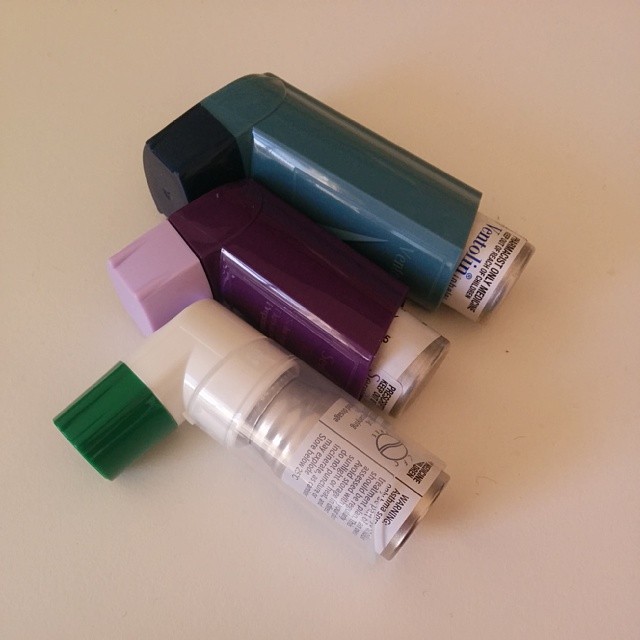The photograph captures a top-down view of three inhalers aligned vertically on a tan or off-color brown surface. The inhaler at the top features a dark blue and black cover with a medication canister labeled "Ventolin" in blue letters, and a cautionary label above warning "pharmacist only medicine keep out of reach of children" in black letters. Below it is a second inhaler, characterized by its dark purple body with a light purple cap. The third inhaler, positioned at the bottom, has a white base with a green cap, and a clear plastic section revealing the attached medication canister. All three inhalers represent modern designs, with the blue and purple inhalers appearing particularly up-to-date, while the green-capped inhaler does not have a cover over the medication canister, making it clearly visible.